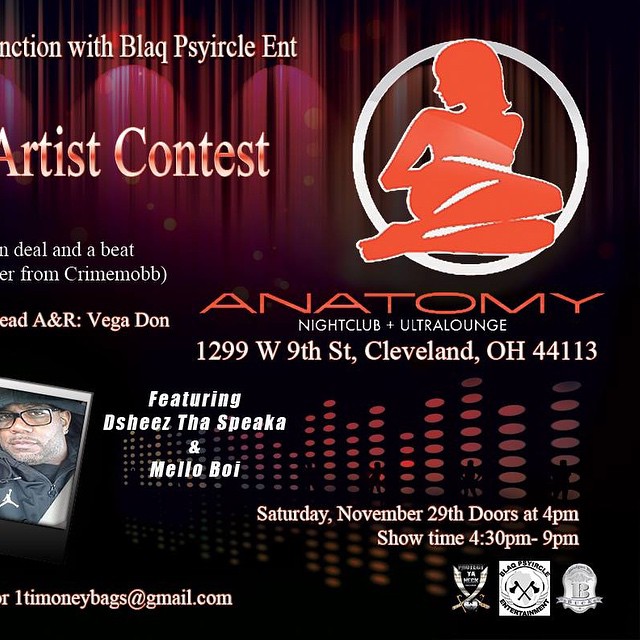This image is an event advertisement with a dark, blackish-reddish background and white and red text. The top prominently features the text "Black Circle Ent Artist Contest," and on the right side, there's a logo of a cartoonish, provocative lady looking right, depicted in a red silhouette. The ad provides details about the event, including a prominent entry, "Deal in a Beat from Crime Mob Lead A&R Vega Dawn," and the venue, "Anatomy Nightclub Ultra Lounge, 1299 W 9th St, Cleveland, OH 44113." A picture of a Black man, likely one of the performers, appears on the left side of the ad. The names "Dashis the Speaka" and "Mellow Boy" are highlighted as featured performers. The event is scheduled for Saturday, November 29th, with doors opening at 4 pm and the show running from 4:30 pm to 9 pm. An email contact, 1timoneybags@gmail.com, is listed for further inquiries. The bottom right of the ad contains three small, somewhat indistinct logos. The overall style of the ad indicates it's for a nightclub event, possibly a contest, with vivid usage of red, black, and white colors to draw attention. The image seems designed to appeal to a nightlife audience, blending graphical elements with informative text.